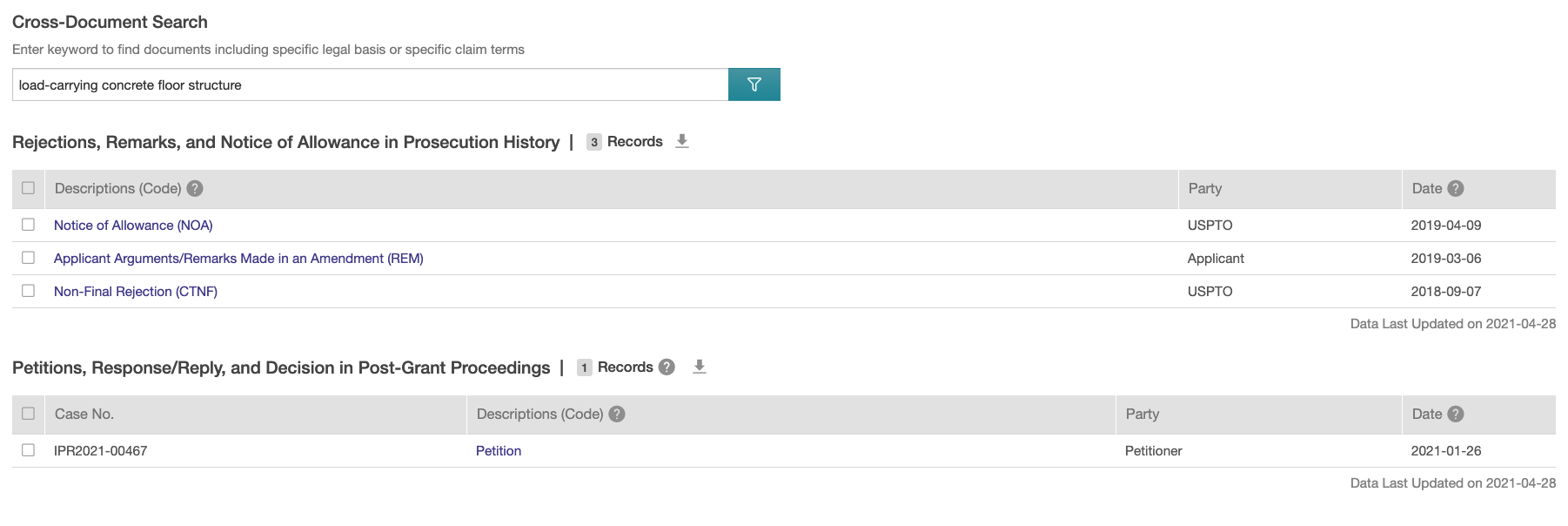The image showcases a user interface of a computer application or website, featuring a clean and structured layout. At the top is a header with bold, left-aligned black text on a white background reading "Cross Document Search." Directly beneath, a smaller font provides instructions: "Enter keyword to find documents including specific legal basis or specific claim terms." Below this, occupying approximately 45% of the screen's width, is a horizontal search bar. Inside the search bar, the text "load carrying concrete floor structure" is typed. Adjacent to the search bar is a teal-colored search button, symbolized by an inverted funnel icon.

Underneath this section, on the left side, bold and slightly larger text reads "Rejections, Remarks, and Notice of Allowance in Prosecution History." To the right of this text, there is the number "3" followed by the word "records," accompanied by a download icon. Below these elements, the interface displays a list of search results, each with an unselected checkbox to the left, indicating that multiple selections can be made.